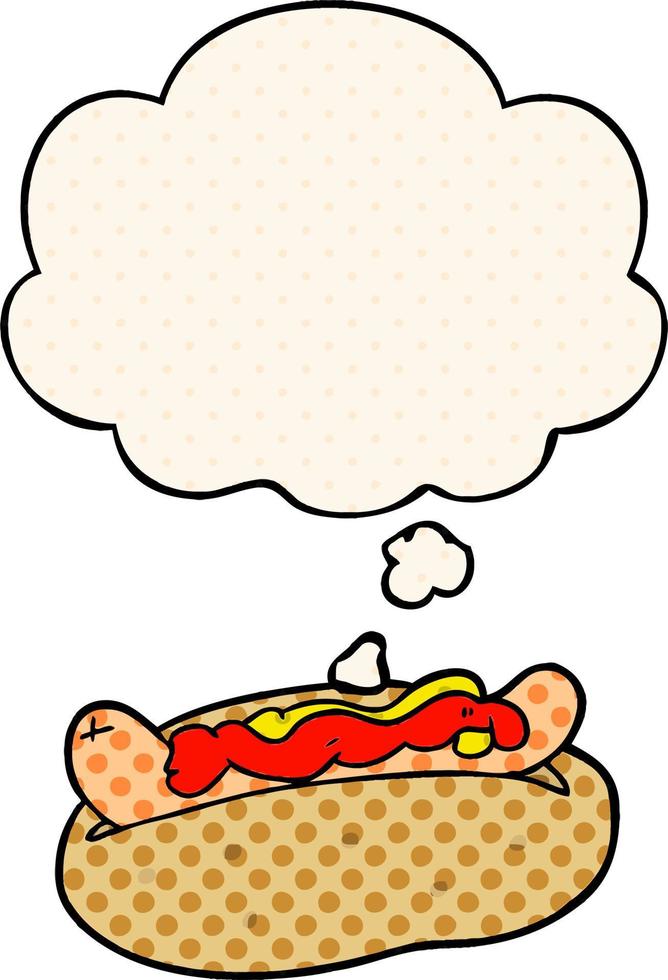This image is a colorful, cartoon-style depiction of a hot dog nestled in a bun. The bun is tan with darker brown polka dots, giving it a playful, retro feel reminiscent of 1950s cartoons. The hot dog itself is a pale peach color, also adorned with darker tan spots. It features generous swirls of red ketchup and yellow mustard. Rising above the hot dog is a thought bubble, similar to those found in comic strips, intended to convey the character's thoughts. This thought bubble is white or a light cream color and is also patterned with smaller, darker polka dots, though the pattern is subtler. The thought bubble, like a nod to Roy Lichtenstein's art, remains blank, leaving the hot dog's thoughts a mystery.